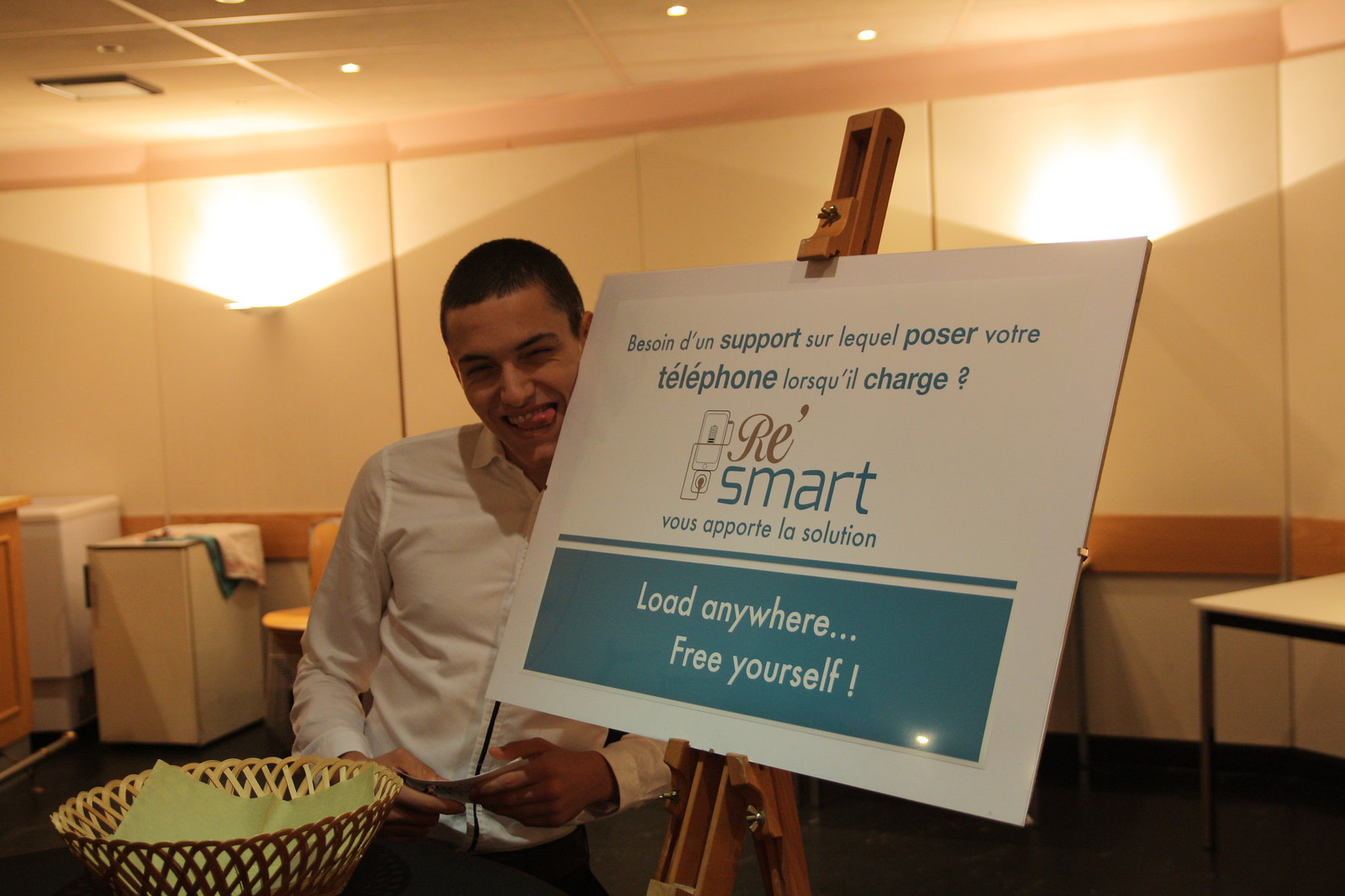In the center of this indoor setting, a young man with very short black hair is dressed in a white button-up shirt tucked into black pants. He stands confidently, holding a card or note in his hands, while making a playful expression with his tongue slightly out and squinting at the camera. To his right, a brown easel holds a white sign with text predominantly in another language, including phrases like "Boisson, Don, Support sur, Laquel poser votre téléphone lorsqu'il charge," and "Ray Smart, Rouse La Porte La Solution." The bottom of the sign reads "Load Anywhere, Free Yourself." The room, likely a conference or presentation setting, features light cream-colored walls, ceiling-mounted lights, and is sparsely furnished with tables, chairs, and a basket with a green paper napkin in the bottom left corner. The background includes decks and cabinets, enhancing the formal ambiance of the event.